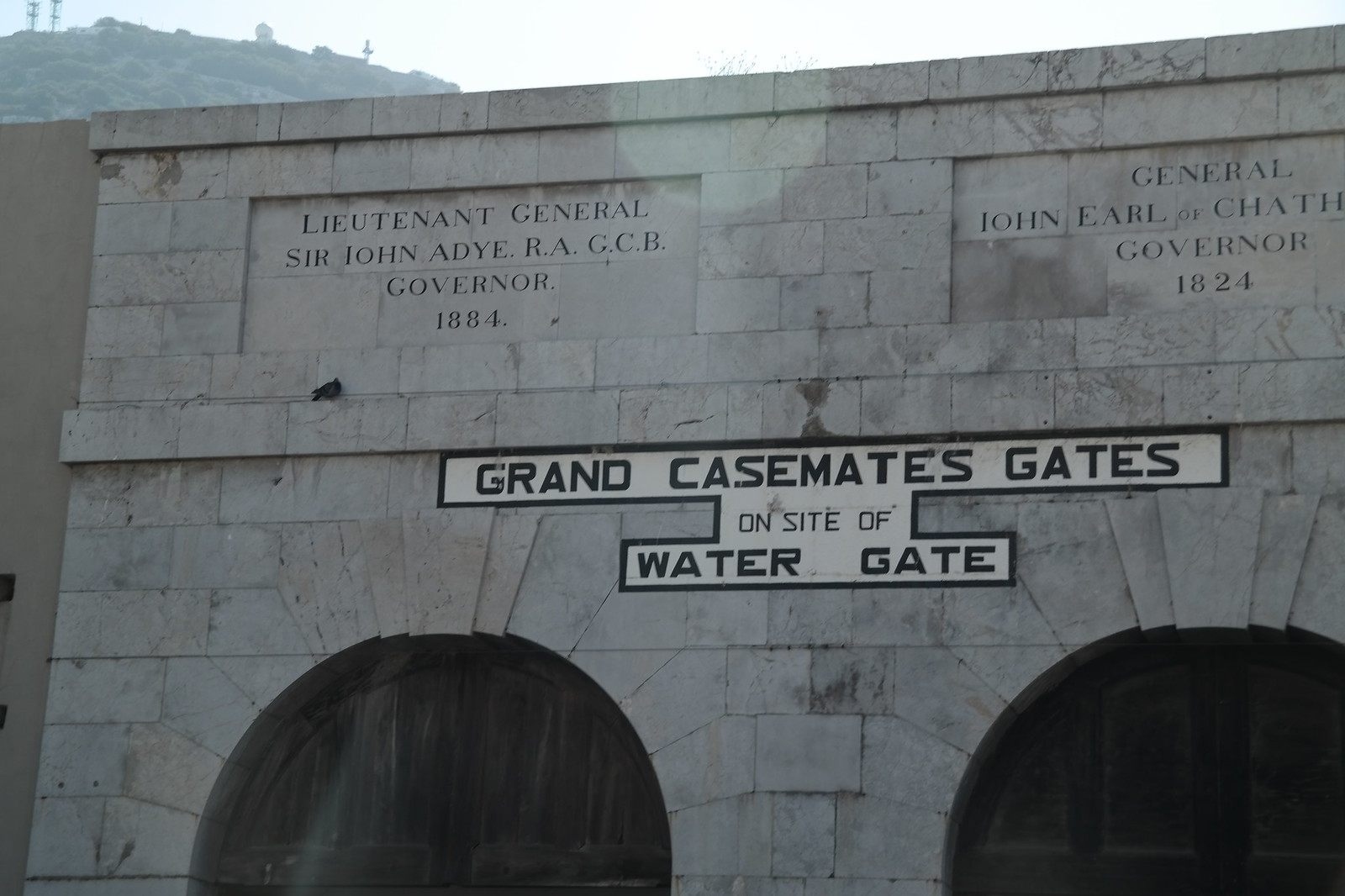The image displays a historical stone structure, primarily featuring two arched tunnels at its base, each topped with black doors. Prominently displayed above the tunnels is an inscription in bold uppercase letters: "Grand Casemates Gates on Site of Watergate." Set against a backdrop of a steep, mountainous area dotted with buildings and trees, this outdoor scene is illuminated by natural white light. Additional engravings on the structure include the names and titles of two past governors: on the left, "Lieutenant General Sir John Adye, R.A.G.C.B., Governor 1884," and on the right, although partially obscured, likely reads, "General John, Earl of Chatham, Governor 1824." The stone used appears to be large gray bricks, giving the structure an old-fashioned, fortified look.